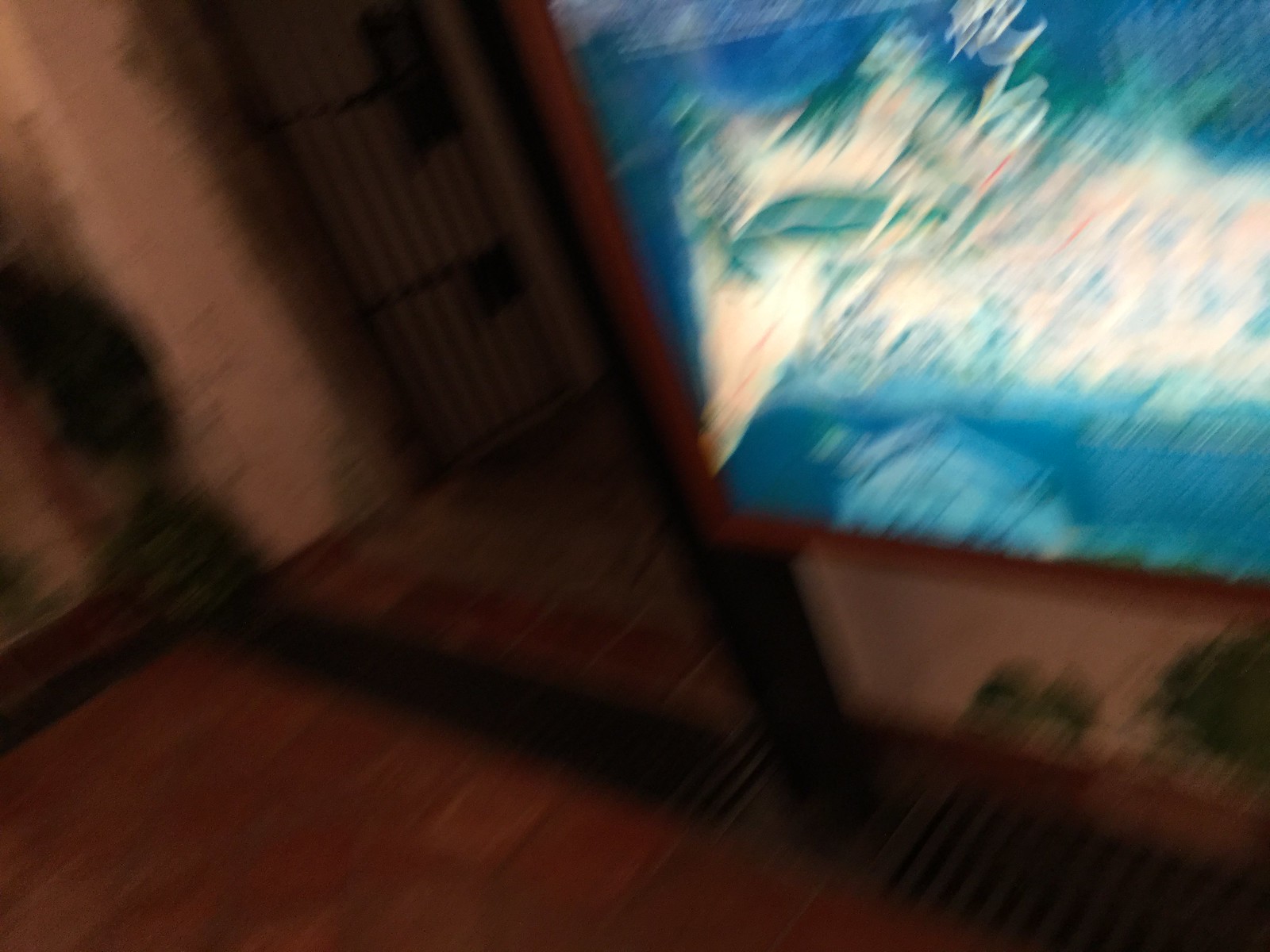This photograph captures the entrance to a building from an unusual angle, presenting a somewhat chaotic scene due to its blurriness. The focus appears to be on a black iron gate to the left, which is open and leads into a corridor with square tiles or bricks on the ground. The right side of the photo features a brightly illuminated sign or picture, set within a brown frame, which might be a television or a large aquarium with indistinct blue, green, and white imagery. Below this illuminated section is a wooden frame displaying a tan wallpaper with hints of tree tops painted on it. Additionally, there are two noticeable grates on the floor, one stretching across the image and another parallel to it, both possibly for drainage. On the far right, slightly obscured by darkness, is a white door with black vertical and horizontal bars, leading into what seems to be another section or a separate hallway. Throughout the image are scattered elements like green shrubs and a small patch of green grass, giving a slightly cluttered and indistinct overall view.